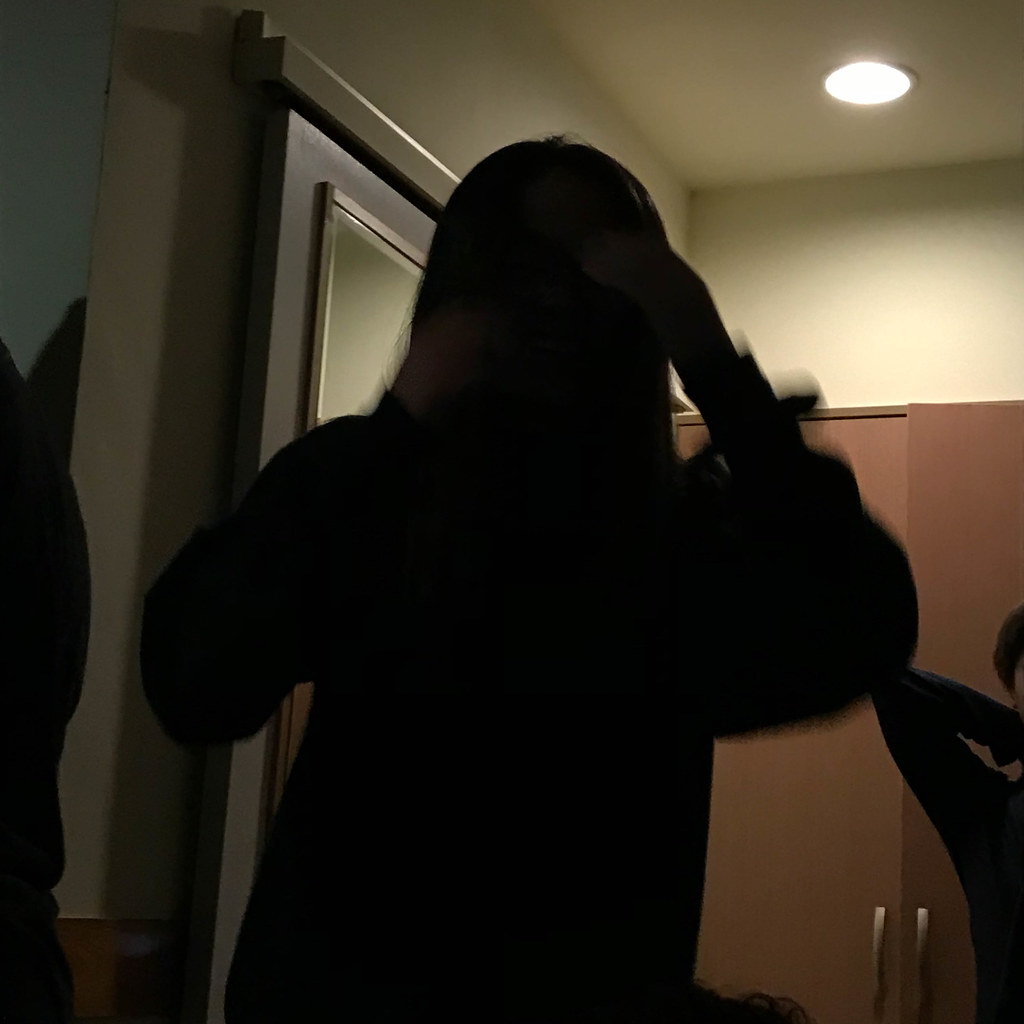The photograph captures an indoor nighttime scene, likely in a bedroom, illuminated by a single artificial light source positioned near the top of the frame. The focus is on two shadowed figures, suggesting they might be children or teenagers. The main subject stands obscured in darkness; their long hair concealing their face completely. They are dressed in dark clothing, with both arms raised. In the background, there is a wooden wardrobe painted blue and reflecting light from a nearby mirror, adding depth to the space. At the bottom edge of the image, another person, possibly a teenage boy, is partially visible with one arm bent at a right angle, resembling a "chicken wing" pose. The scene conveys an atmosphere of casual, playful interaction among the kids, captured in the shadows and artificial light of a cozy bedroom.